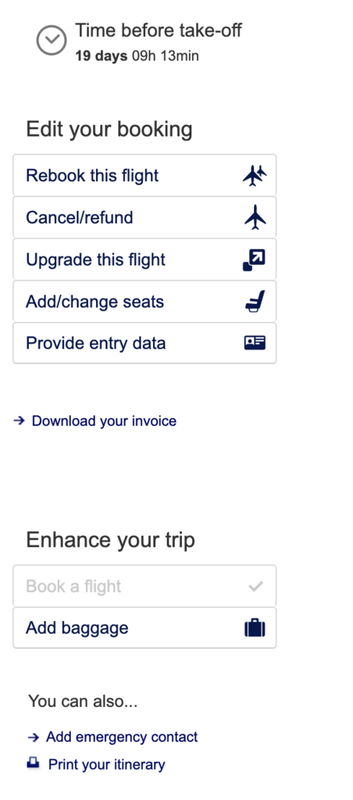This is a screenshot taken on a cell phone from an app where a flight has been booked. The background is white, and at the very top in black lettering, it displays: "Time before takeoff: 19 days, 9 hours, 13 minutes." To the left of this text, there's a black circle with a white checkmark inside. 

Below that, the screen features a section labeled "Edit your booking" with several actionable links:

1. "Rebook this flight" accompanied by an icon of two planes on the right.
2. "Cancel/Refund" with an icon of a single plane.
3. "Upgrade this flight," indicated by an arrow in a black box pointing to the upper right corner.
4. "Add/Change seats," alongside an icon of a plane seat.
5. "Provide entry data," with an icon of an ID card.

Further down, there is a link to "Download your invoice." 

Underneath this link, a section titled "Enhance your trip" appears. The first item here is "Book a flight," which shows a checkmark in light gray, indicating that the flight has already been booked. Below this, in black lettering, it says "Add baggage" with a suitcase icon on the right. 

The final section reads, "You can also," followed by two links: "Add emergency contact" and "Print your itinerary."